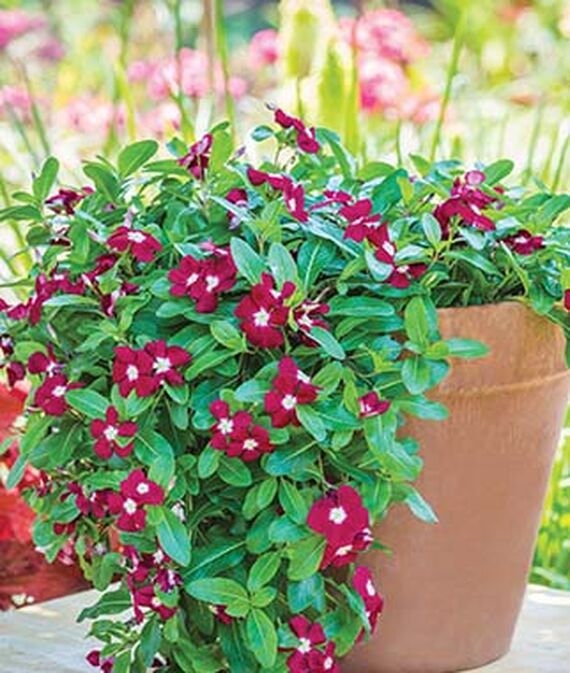This close-up image captures a charming terracotta pot brimming with a lush green myrtle plant cascading over its left side. The focal point is a vivid reddish-pink flower with a pristine white center, gracefully extending from the plant. The terracotta pot, marked with subtle water stains, sits prominently on a gray, cement-like table surface. In the blurred background, tall pink flowers emerge, adding height and depth to the scene. Adjacent to the pot, subtle hints of additional greenery and a mysterious red object enhance the composition, making it evident that the setting could be a porch or patio overlooking a flower garden.